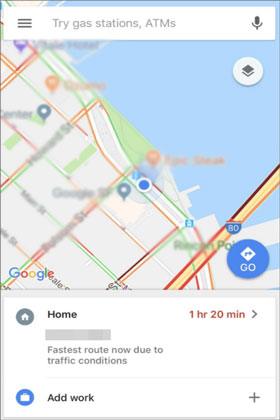This image appears to be a screenshot of a web page displaying mapped directions obtained from a Google search. 

At the top of the page, a map is prominently displayed with its titles blurred out. Running horizontally across the top of the map is a white search bar. On the left side of this search bar, three stacked black bars (a menu icon) are visible, followed by the text in black: "Try Gas Stations, ATMs" with "ATMs" capitalized partially – only the letters A, T, and M are in uppercase, and the 's' is in lowercase. On the far right side of the search bar, there is a black microphone icon.

Directly underneath the microphone icon, but outside the search bar and superimposed over the map, is a small white circle containing a black diamond shape. 

In the bottom right-hand corner of the map is a blue circular button displaying a white diamond with a blue triangle pointing left. Below this, the word "Go" is written in white text.

At the bottom of the map, a white information box appears. In the upper left corner of this box is a black circle with a white home icon, followed by the word "Home". On the opposite side of this box, in red text, it states, "1 hour 20 minutes" next to a small black right-pointing arrow icon. Below this, there is a small gray bar with the text, "Fastest route now due to traffic conditions," followed by another small gray dividing line separating this information from a secondary box.

In this secondary box, on the left side, a blue circle shows a white briefcase icon. Beside this icon, the text reads "add work" in black. To the right of this text, there is a small black plus symbol near the right edge of the box.